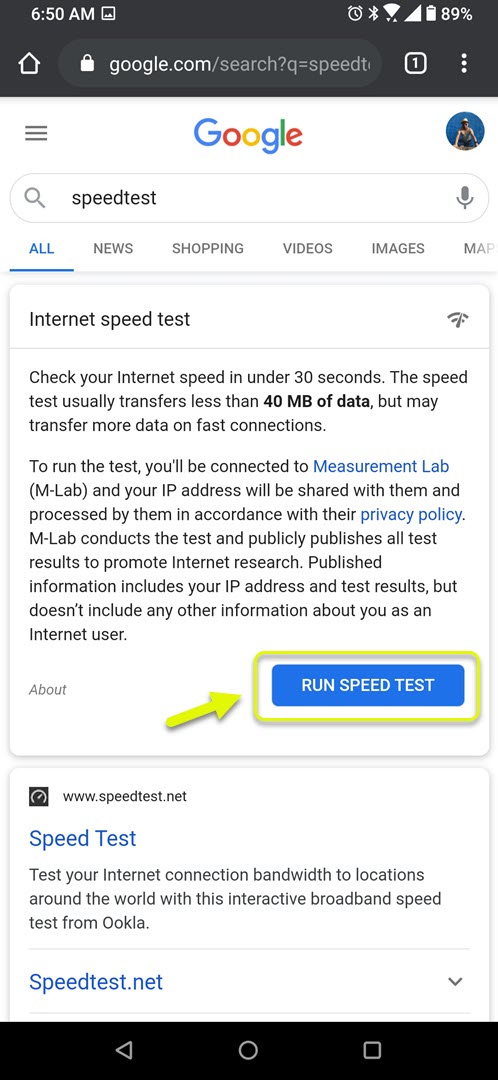This is a detailed screenshot from a smartphone displaying a Google search result for "speed test" at 6:50 AM. The status bar at the top of the screen shows common icons such as signal strength, Wi-Fi, and a battery level at 89%. Just below the URL bar indicating a Google search, there's prominently visible text about the internet speed test. 

The description notes: "Internet speed test. Check your internet speed in under 30 seconds. The speed test usually transfers less than 40 megabytes of data, but may transfer more data on fast connections. To run the test, you'll be connected to Measurement Lab (MLab), and your IP address will be shared with them and processed by them in accordance with their privacy policy. MLab conducts the test and publicly publishes all test results to promote internet research. Published information includes your IP address and test results, but doesn't include any other information about you as an internet user."

There's a highlighted section with a circled "Run Speed Test" button accompanied by an arrow pointing towards it, emphasizing the next action. Below this section, there’s a reference to "speedtest.net," mentioning it provides an interactive broadband speed test, allowing users to test their internet connection bandwidth to various locations around the world. Additional navigation buttons at the bottom of the browser are visible, providing options such as going back.